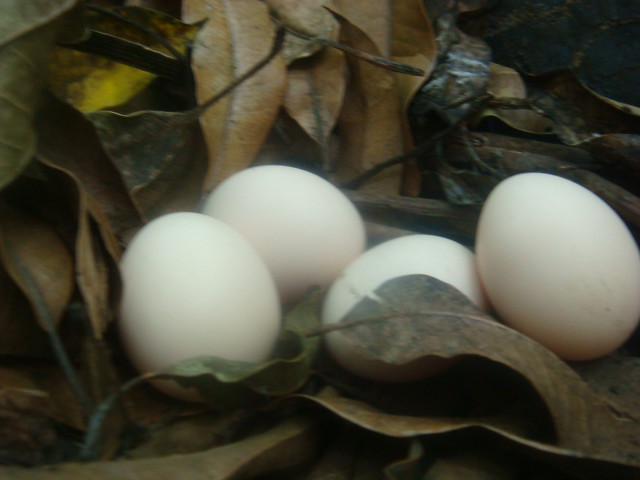This slightly blurry and grainy rectangular photograph captures a cluster of four white eggs haphazardly nestled amongst a variety of decaying leaves scattered across the ground. Each leaf varies in size and color, with some being twice the length of an egg. The leaves display an array of hues—dusty brown with dark dirt streaks, yellowish tones, dark green possibly due to mold, and even deep black. Some leaves are smooth and teardrop-shaped, while others are curled and crumpled. Notably, three long, smooth, very brown leaves dominate the top center area, contrasting with the very black and dirt-covered leaves in the top right corner. Light brown leaves with visible stem veins and a wavy outline occupy the bottom left corner, while a living, windy green leaf appears in the same area. In the bottom left corner, a tiny blue stalk adds a hint of color variation. The four eggs are positioned in the middle of this leaf tapestry: two lying close together on the left, one centered but slightly turned away, and one standing up slightly on the right.